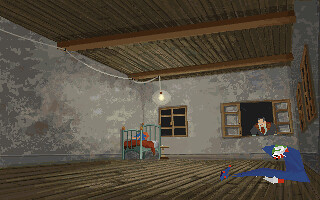This detailed image presents a watercolor painting of a simple, almost barren, indoor scene that resembles an environment from a video game. The room, made of concrete walls and featuring a wooden floor, has a twin bed positioned in the upper corner against the back wall. Above the bed hangs a small light bulb from the wooden ceiling, which is reinforced with two large horizontal beams. The setting includes two windows: one directly behind the bed, consisting of six small panes separated by brown frames, and the other on the left side, depicted as open. Peering through this open window is a man with short hair, dressed in a suit and tie, a gray jacket, and a white shirt.

In the foreground, sitting with his legs stretched out towards the right, is a forlorn clown dressed in a blue suit and hat. The clown's head is bowed down, his face painted white, with a distinctive red nose, red highlights on his shoes, and collar. The overall atmosphere is accentuated by the sparse furnishings and the muted colors of the scene, creating a melancholic, almost eerie ambiance.